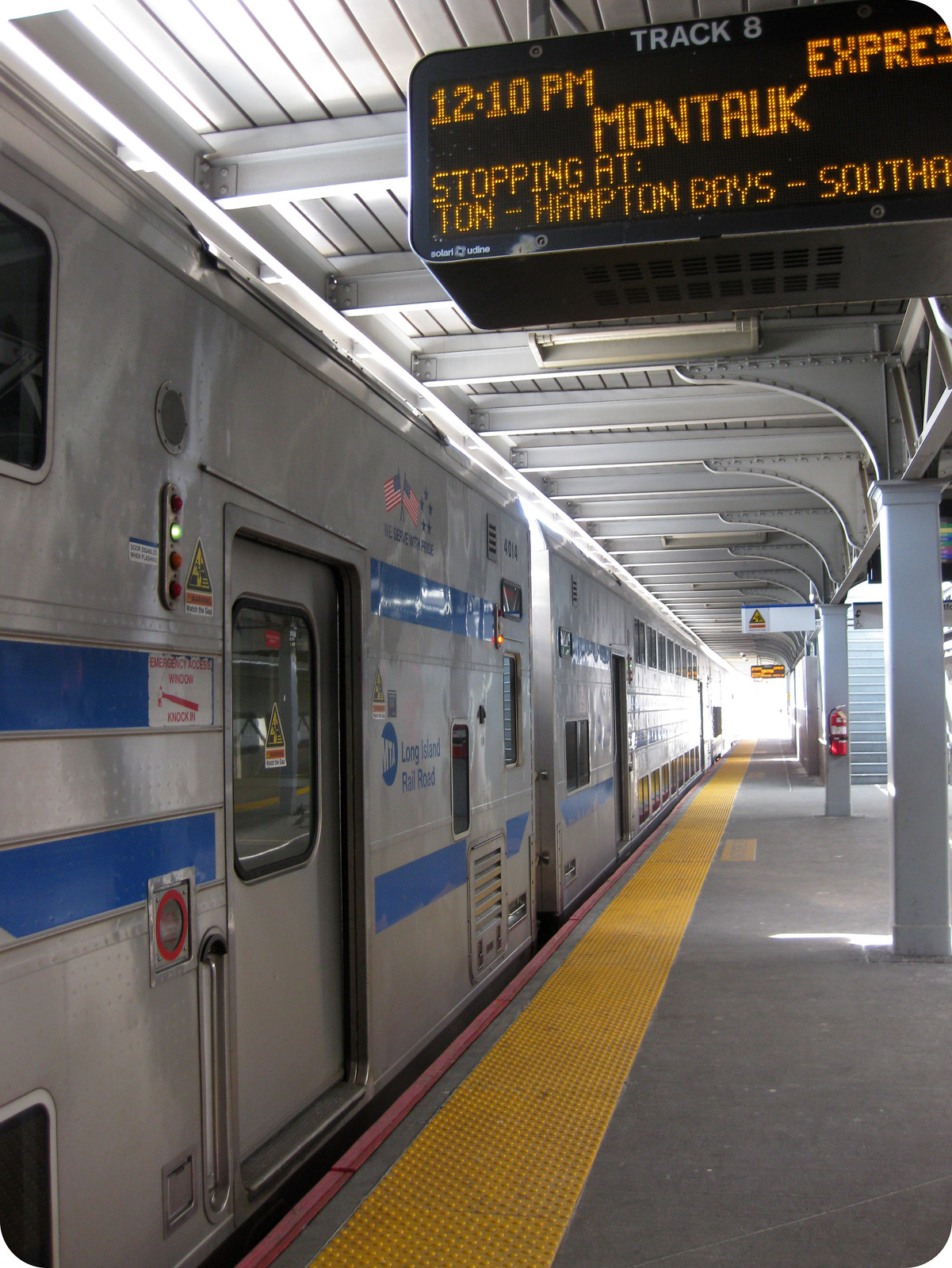This detailed image depicts a sunny day at an outdoor train station platform, where a sleek, silver train adorned with blue stripes stands parked. The train, consisting of multiple two-story cars, is protected by a metal canopy that shields the platform from the weather. The grey platform features a prominent yellow caution bar, warning passengers to stay behind it until the train has stopped. There are several pillars along the platform, one of which supports a red fire extinguisher. Atop another pillar, a well-lit scoreboard informs travelers that the current time is 12:10 PM and that the express train to Montauk, stopping at Townhampton Bays and Southampton, is on track 8. The platform is devoid of passengers and the doors of the train are closed, contributing to the serene and orderly atmosphere of the scene.